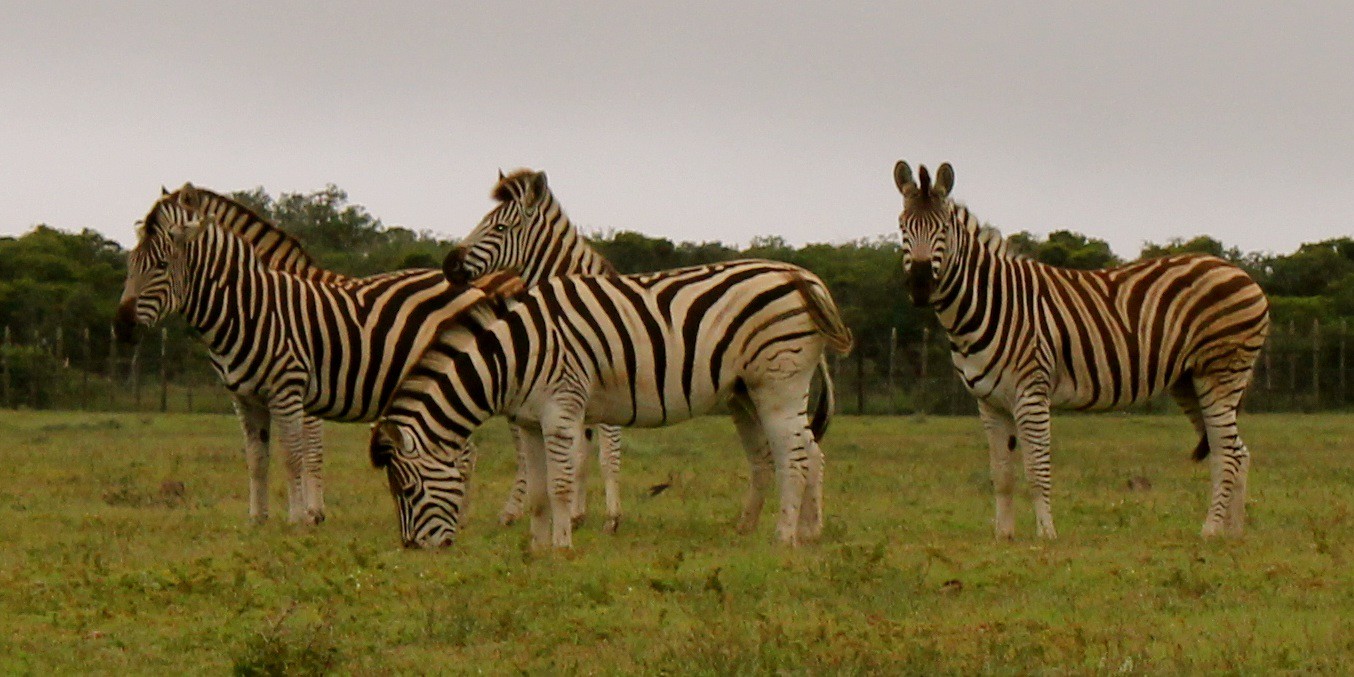This detailed image captures a vivid scene of four zebras standing in a grassy field. The zebras, each with their distinctive black and white stripes, populate the foreground with one central zebra bending down, head lowered as it grazes on the grass. This central zebra appears to have some orangish dirt stains on its fur. To the right of this zebra, another zebra with similarly stained fur stands closely, its head turned to directly face the camera and revealing a dark brown texture on its back. Behind the grazing zebra, a third zebra's head peeks out, looking to the left, partially obscured by the central figure. The fourth zebra, positioned farthest to the left, is distinct with its darker stripes and slightly orange mane, facing left and gazing off into the distance. The backdrop consists of a tree line enclosing the field, interspersed with patches of fencing, under a stormy sky that is bleached white and gray, suggesting impending rain. The grassfield itself is a mix of green and yellowish tones, reflecting the natural wear of the landscape. Overall, the composition conveys a serene moment in a nature preserve or zoo-like setting, with each zebra's presence adding depth and character to the scene.